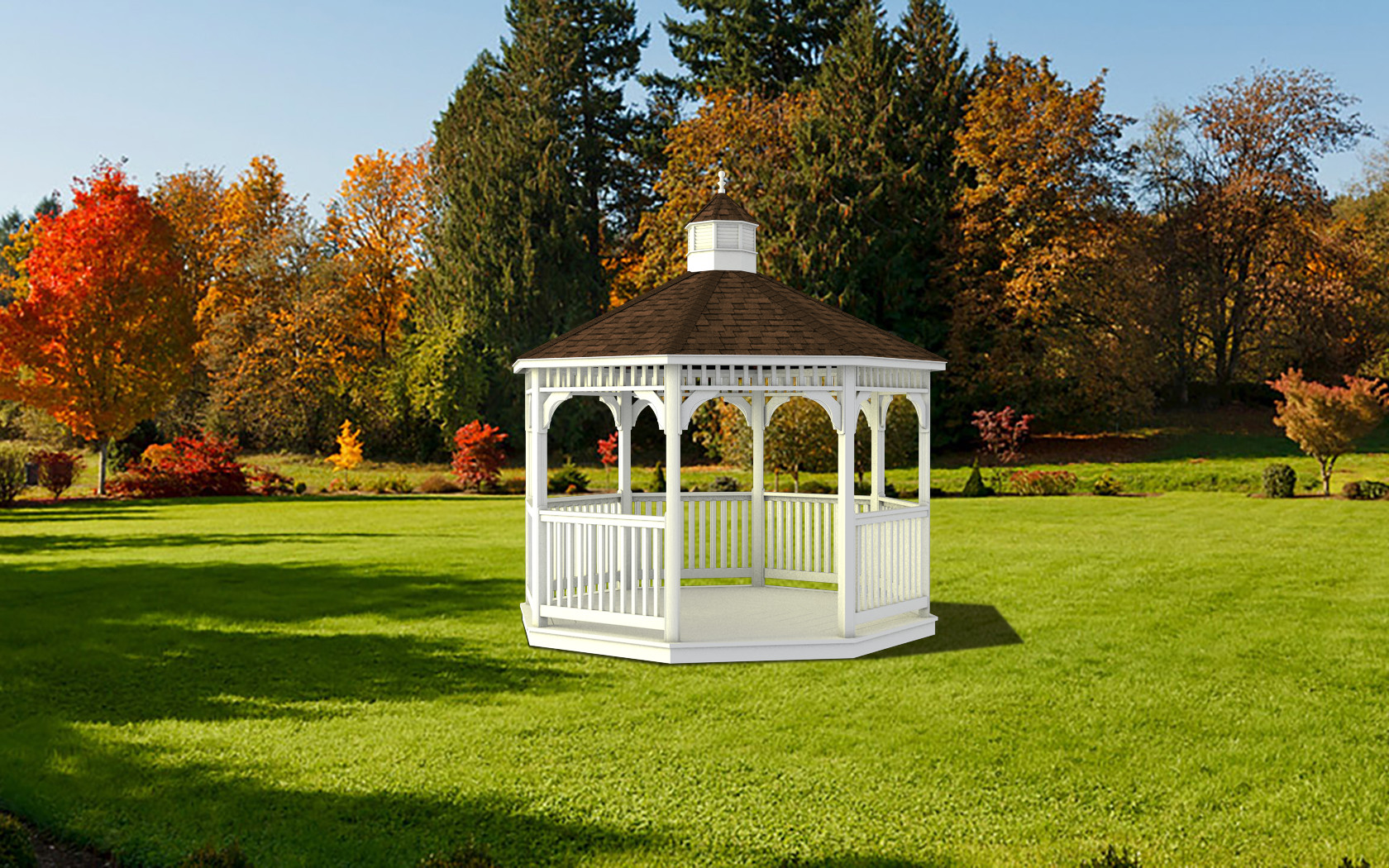This photograph captures a serene autumn landscape featuring a white octagon-shaped gazebo with a distinctive conical roof adorned with brown shingles. Positioned centrally in a meticulously mowed, lush green lawn, the gazebo stands without any seating or furniture inside. The expansive grassy area is surrounded by thoughtfully arranged landscaping, including smaller bushes and shrubs. In the distance, towering evergreen trees retain their dark green hue, while a medley of large deciduous trees exhibits a vibrant display of fall colors, with leaves transitioning through shades of red, gold, orange, and yellow, alongside some that remain green. The sky overhead is a pale blue, adding to the image's bright and sunny ambiance.